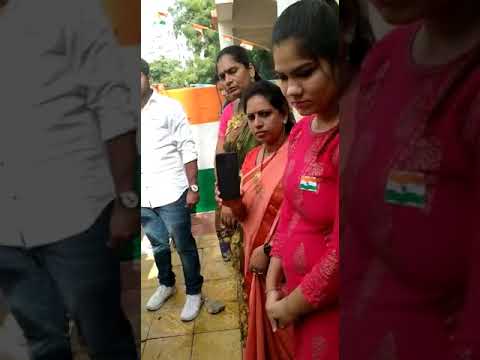In the center of the image, four brown-skinned women stand in a line, all wearing traditional, vibrant Indian dresses with darker sashes draped over their shoulders. The first woman on the right, in a pink dress, looks downward. The second woman, also in a pink dress with a lighter pink sari wrap, gazes directly at the camera while holding a black cell phone towards us. The third woman wears a brighter pink dress with a brown sari sash, and she, like the first, looks downward. Only a portion of the fourth woman's face is visible as she, too, looks downward. Their dark brown hair is all pulled back.

On the left side of the image, a man in a white shirt with rolled-up sleeves, blue jeans, and white shoes stands, though his face is out of the frame. He appears partially in an enlarged and darkened backdrop that extends to both sides of the central image. This backdrop also includes an enlarged, darkened version of the first woman in pink on the right third of the picture. The scene is set against a yellowish, square stone-tiled floor with some greenery and a building faintly visible in the background, creating a stark, solemn mood among the otherwise brightly dressed women.